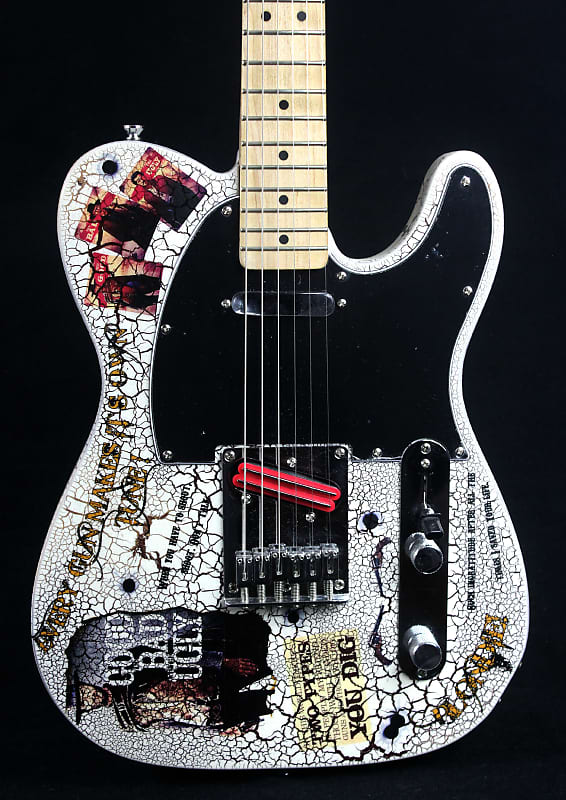This detailed image showcases a close-up of a white electric guitar with a distinctive crackled paint finish, displaying black crackles with white interiors. The guitar is positioned centrally against a black background, with the natural wood-colored fretboard visible at the top right. Notable features include a red pickup in the middle, likely an aftermarket addition. The top left of the guitar body features three small, indistinct magazine cover images, possibly of horror movie characters such as Freddy Krueger, Michael Myers, or Jason. Yellow text on the left side reads "Every gun makes its own tune," accompanied by smaller black text underneath stating, "When you have to shoot, shoot, don't talk." The phrase "Good, Bad, Ugly" appears at the bottom left, alongside more text that is difficult to discern. The presence of various colors such as tan, black, white, and red, along with additional stickers and red bars under the strings, adds to the visually rich and detailed presentation.